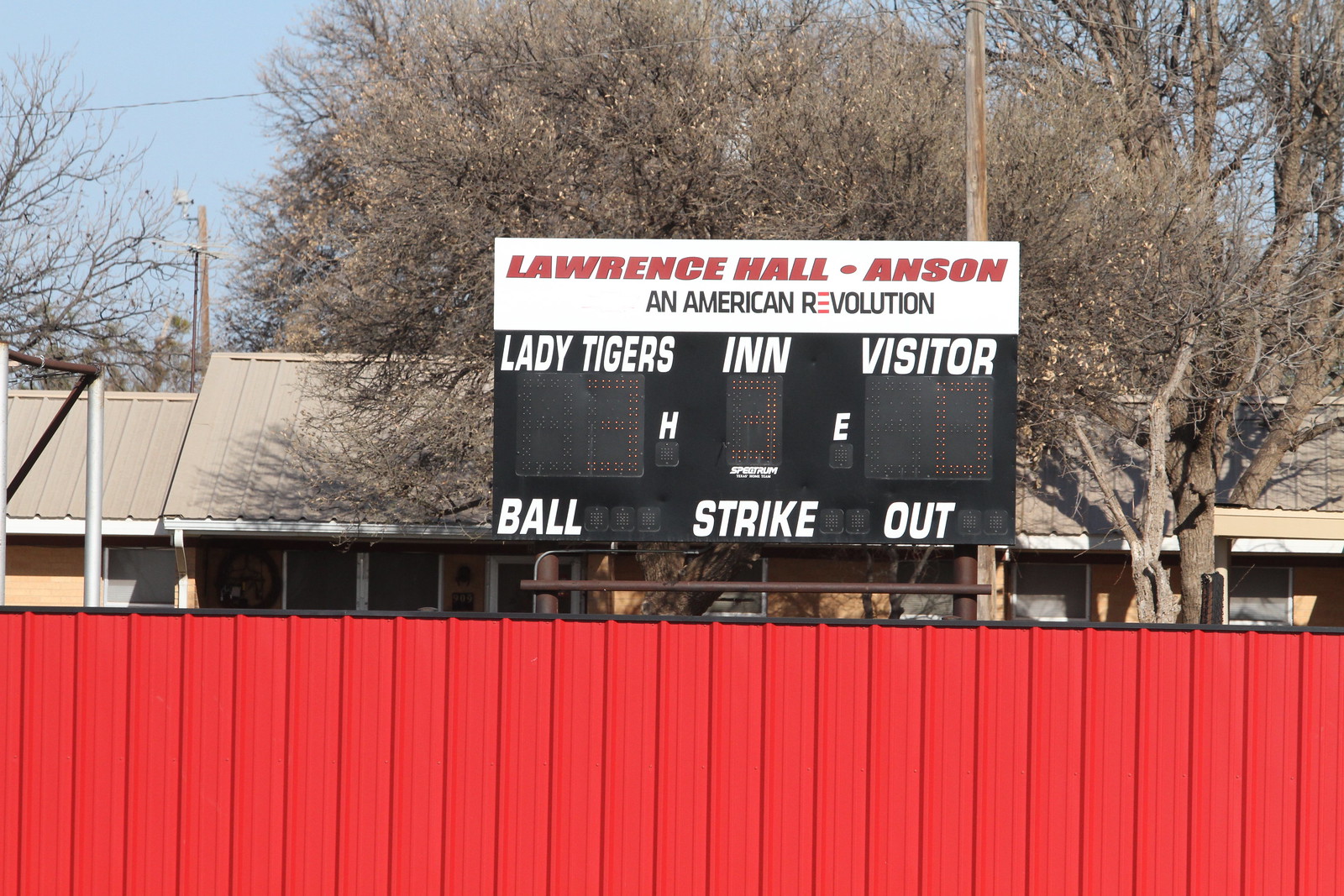The image captures the outfield of a baseball field, dominated by a striking red wooden wall comprised of wooden slats. Mounted above the wall is a black scoreboard with a white banner displaying "Lawrence Hall, Anson, and American Revolution" in red lettering. The scoreboard is divided into sections for "Lady Tigers," the inning, and "Visitor," each with LED screens designated to show scores, currently displaying Lady Tigers 3, inning 3, and Visitor 0. Below these, the sections for "Ball," "Strike," and "Out" are present but not lit up, indicating they are currently off. Behind the scoreboard, there is a house with yellow walls, windows, and a metal corrugated roof, flanked by leafless trees, suggesting it is fall. The entire scene is bathed in bright sunlight, and additional details in the background include a pole, adding context to the setting. The focus on the scoreboard and its detailed features, along with the vibrant, seasonal environment, paints a comprehensive picture of the scene.